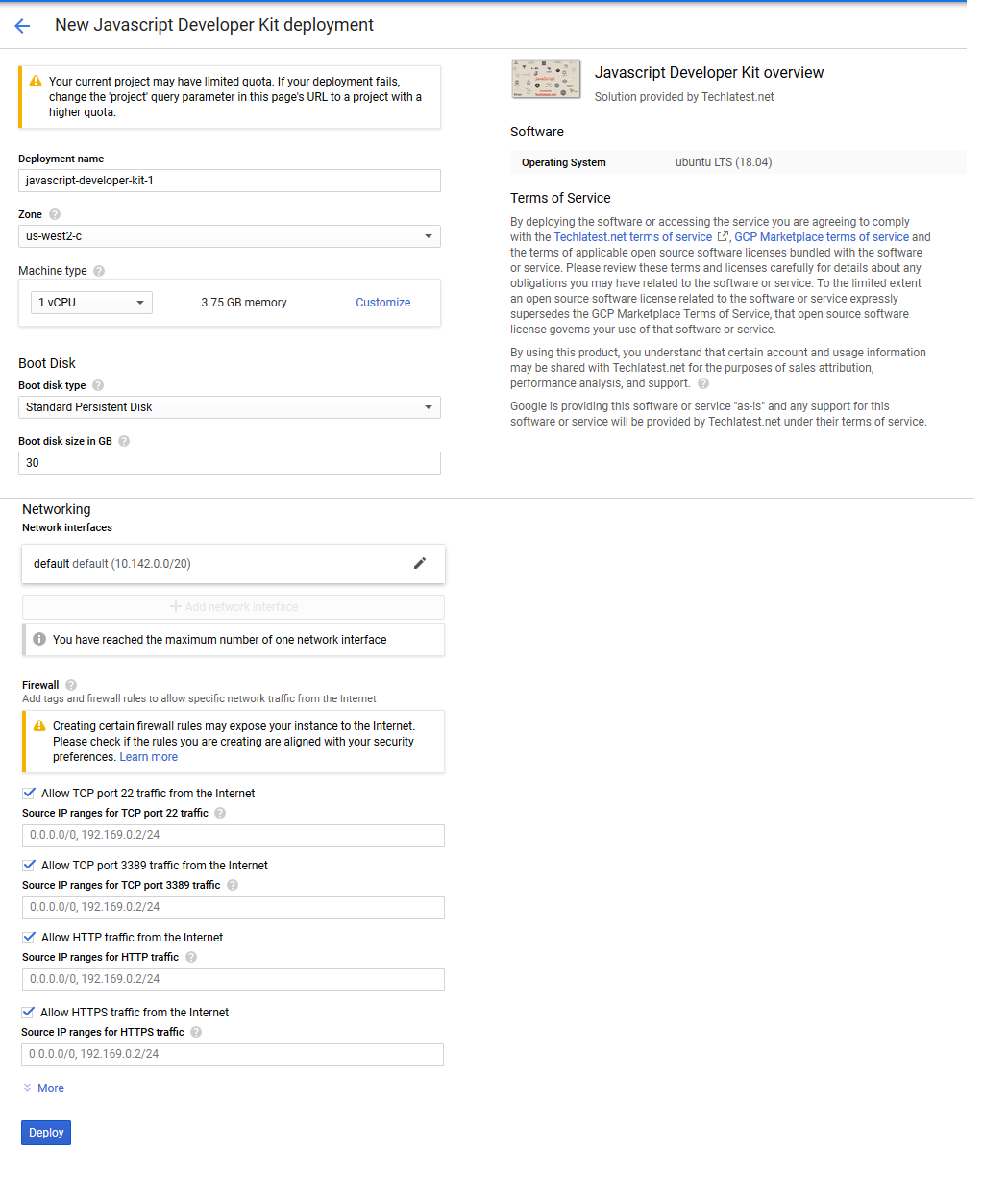**Screenshot of JavaScript Developer Kit Deployment Console**

The screenshot displays a developer console for deploying a new JavaScript Developer Kit. At the top left corner, there's the heading "New JavaScript Developer Kit Deployment." Directly below, a notification warns: "Your current project may have limited quota. If your deployment fails, change the project query parameter in this page's URL to a project with a higher quota."

Details of the deployment are outlined as follows:

- **Deployment Name**: javascript-developer-kit-1
- **Zone**: us-west-2c
- **Machine Type**: 1 vCPU, 3.75 GB memory
- **Boot Disk**: Standard persistent disk
- **Boot Disk Size**: 30 GB (denoted as ngb-30)
- **Networking**:
  - **Network Interfaces**: Default

On the top right side, the console displays an overview section labeled "JavaScript Developer Kit Overview - Solution provided by techietest.net." The chosen software includes the operating system "Ubuntu LTS (18.04)." 

This comprehensive layout helps developers set up their environment with explicit machine and network configuration details, enhanced by guidance from TechieTest.net.